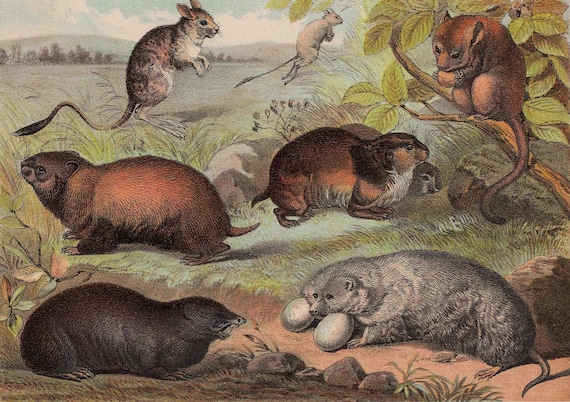In this detailed and colorful painting, seven different marsupial and rodent-type animals are depicted in a fairly realistic style with a palette of washed-out greens, grays, and tans. The setting features an open grassy area that borders a waterway, with a backdrop of rolling hills and a clear daytime sky. In the lower left corner, there is a dark gray shrew-like creature. To its right, in the lower right corner, a fluffy gray rodent or marsupial cradles two eggs near its face. Above these, a collection of marmoset-type rodents is positioned centrally. In the upper section of the image, there are springtail mice hopping like kangaroos to the upper left, while a brown, long-tailed marsupial, possibly resembling a red panda, sits perched on a tree branch. The overall scene is enriched with elements of greenery, including high grasses and sparse trees, creating an impression of a marshland or shoreline.